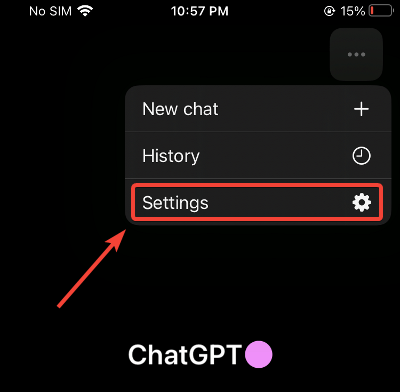This is a detailed screenshot of a settings page on a smartphone with a black background and dark gray elements featuring white text. In the top right corner, there's a dark gray box containing a horizontally-aligned three-dot icon. Below this icon, an opened menu displays three rows of buttons, each with descriptive text on the left and corresponding icons on the right. The first button, labeled "New Chat," has a plus sign icon. The second button, labeled "History," includes a clock icon. The third button, labeled "Settings," is marked with a gear icon and is highlighted by a red box with a red arrow pointing to it.

Directly below the menu, the screen shows "Chat GPT" paired with a pink circle accentuating the section. The overall background remains black, lending to the dark theme of the interface. At the very top of the screenshot, the phone's user interface displays essential status information: the top left corner indicates "No SIM,” the center shows the current time as "10:57 PM," and the top right corner shows that the phone's battery is at 50% capacity.